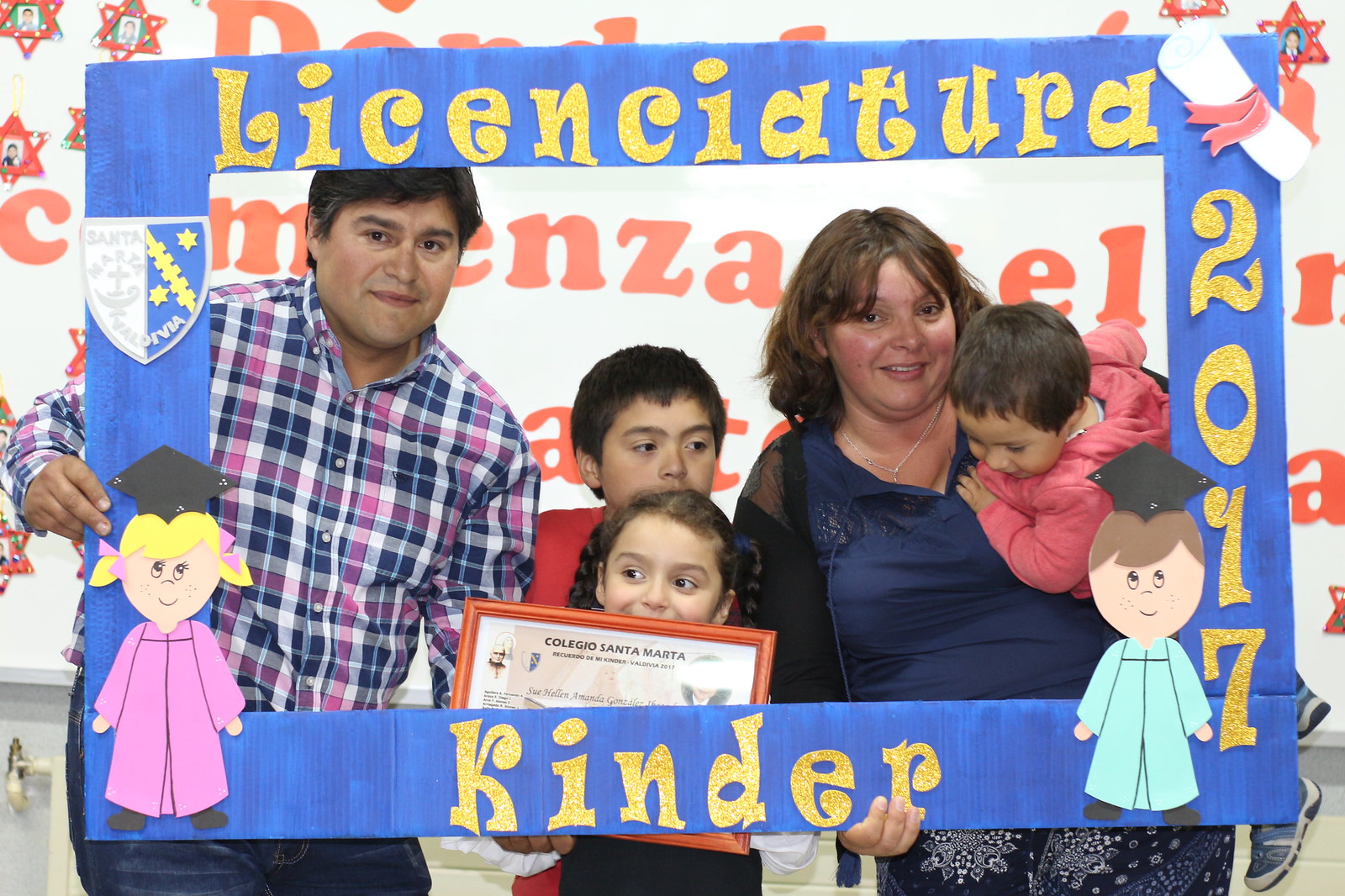The image shows a Hispanic family of five, probably American, posing at what seems to be a celebratory Kindergarten event, likely in California. The family stands in front of a blue photo frame decorated with cartoon characters of a boy and girl in graduation caps. The top of the frame reads "Licenciatura Kinder 2017" in gold construction paper. The father stands on the left, holding up the large blue frame. In the middle, two children—a taller boy and a shorter girl holding a plaque that reads "Colegio Santa Marta"—smile for the camera. The mother, on the right, is holding a toddler. Everyone is smiling, capturing a proud family moment.